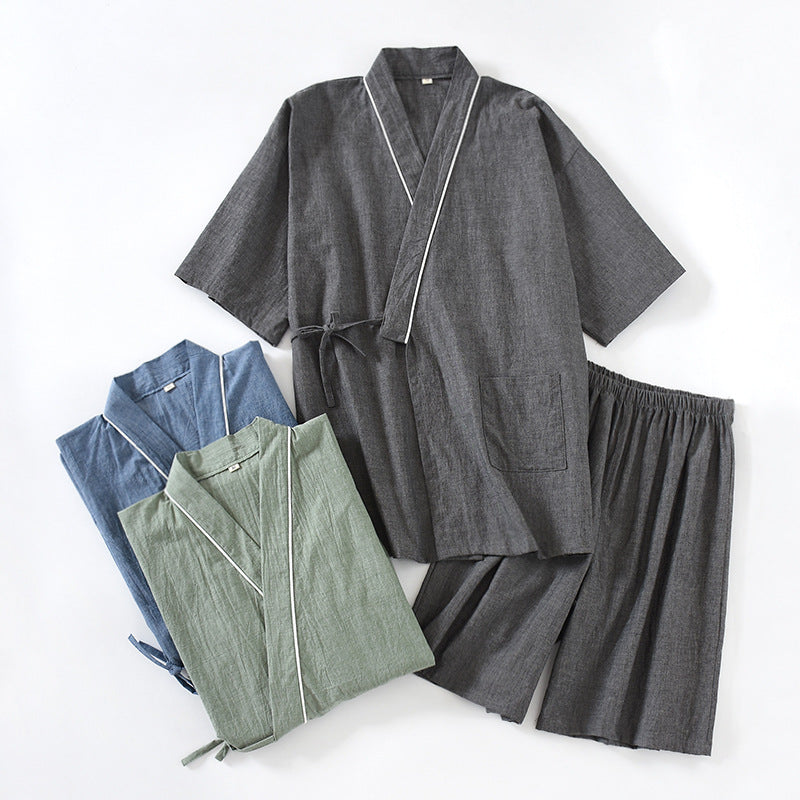This photograph showcases a collection of pajama sets designed in a kimono-wrap style. The primary set is a dark gray ensemble featuring a short-sleeve top with a wrap-around tie that fastens on the side, adorned with white lining around the collar. It includes longer shorts with an elastic waistband, reaching just above the knee. Notably, the top has a practical pocket on the lower left side. Adjacent to the primary set, two additional shirts are visible, neatly folded. One is a sage green while the other is a medium, dusty blue, both echoing the same wrap-around design and white-lined collar as the gray set. These pajama sets, potentially crafted from linen, present a comfortable yet stylish option for both lounging and sleepwear.